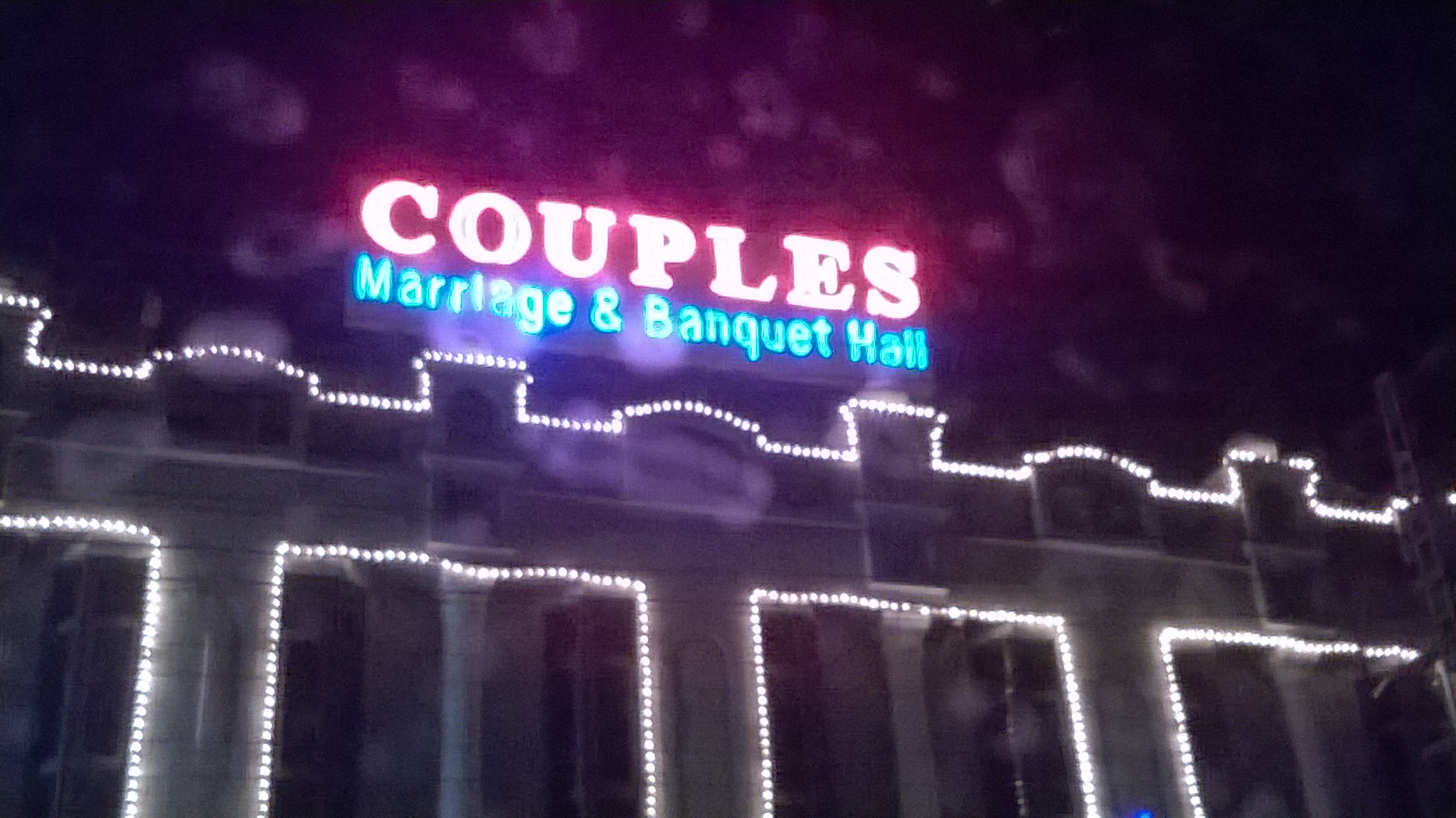This nocturnal image captures the illuminated façade of a building adorned with a colorful sign. The building, photographed at night, features a rectangular frame with the long side extending horizontally. At the top, a vibrant neon sign spells out "Couples" in a blend of pink and orange hues. Directly below, in a striking light blue font, the words "Marriage & Banquet Hall" provide additional context. The ampersand is also in the same light blue shade.

The architectural details of the building are accentuated by white streamlines, which trace the outlines of the structure. These white lights emphasize the pinnacles that rise above the main body of the building, the edges of the roof, and the columns that descend towards the entrance. The illuminated outlines also highlight the portals to the banquet hall, creating a visually engaging and festive appearance. The building itself appears to be white, standing in stark contrast to the pitch-black night sky above, which forms the backdrop of this captivating scene.